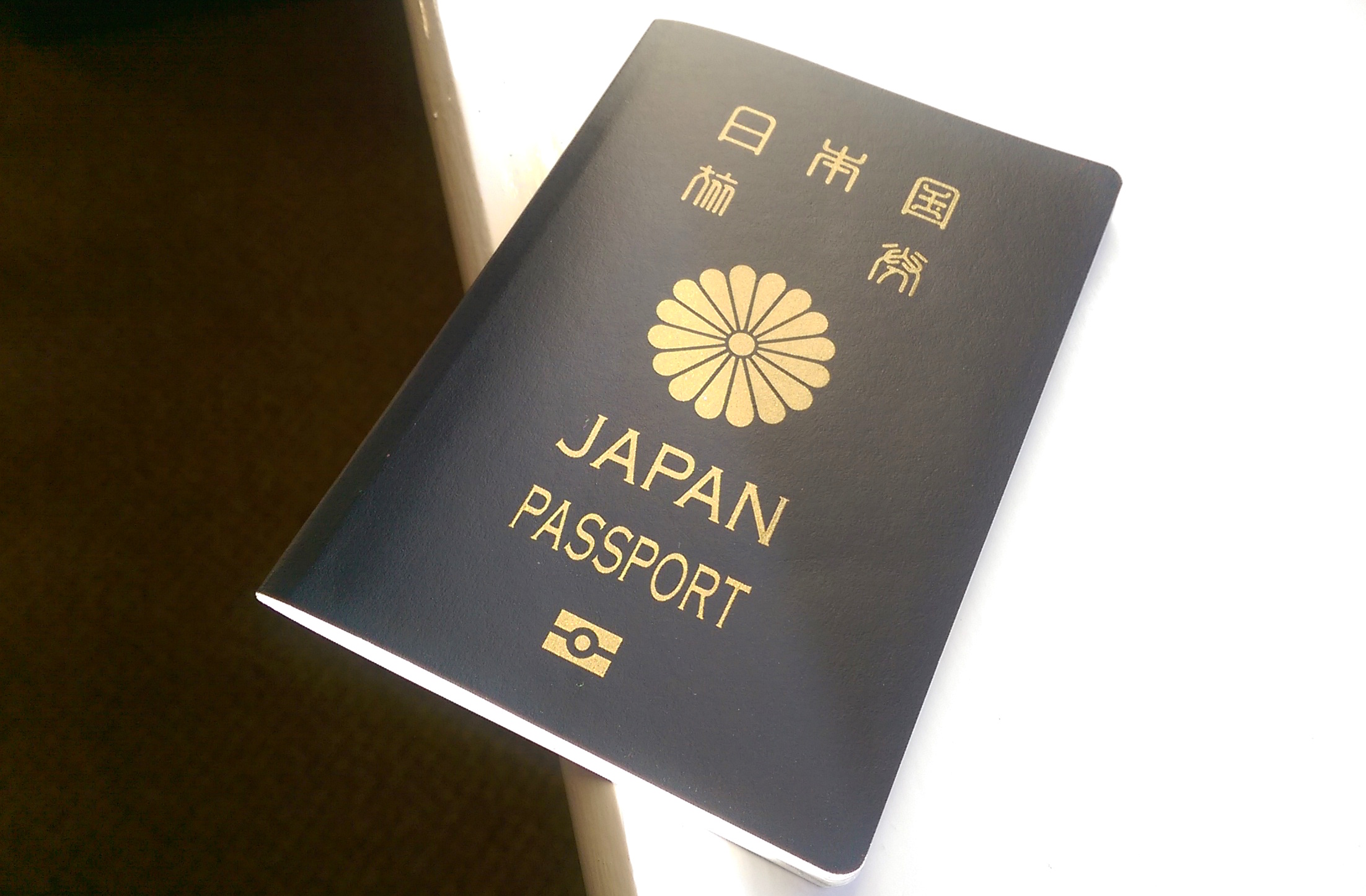This photograph showcases a Japanese passport with a dark cover, either black or dark blue, positioned diagonally at a 45-degree angle on a white desk. The left side of the image hints at a reddish-brown or dark wooden surface. The passport features gold embossed characters and symbols. At the top, there are five Japanese kanji characters. In the center, there's a gold flower with evenly spaced petals radiating from a small circle. Below the flower, the text reads “Japan Passport” in large gold letters. At the bottom, a gold rectangular icon with a line through the middle and a circle, resembling the Japanese flag icon, is depicted. Light reflects off the glossy cover, enhancing its intricate design. The background to the left includes an out-of-focus green carpet.